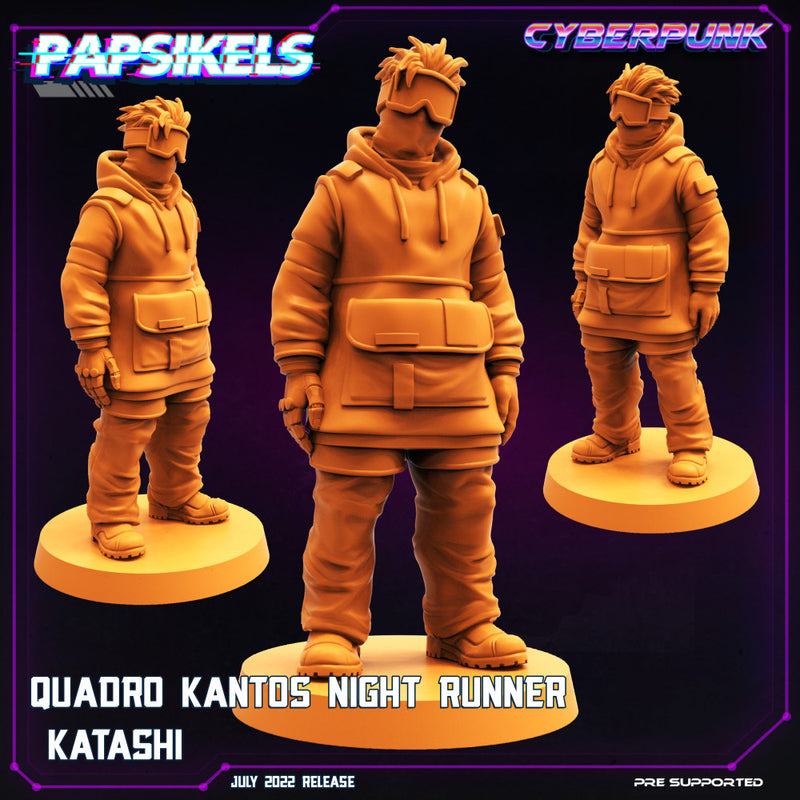This detailed product showcase image is an advertisement for a miniature figurine associated with a Kickstarter campaign. The image prominently features three monochromatic, matte orange 3D renderings of the same character, displayed at different angles—front, right, and left. The character is a male dressed in a bulky hoodie with a spacious front pouch, heavy-duty gloves, regular trousers, and large boots. He sports spiky, loose hair, ski goggles, and a mask covering his face.

In the upper left corner, the image has the distorted, all-caps text "Papsicles" (stylized as P-A-P-S-I-K-E-L-S). The text in the upper right corner says "Cyberpunk," displayed in an italic, bold san-serif font with a gradient that transitions from red to pink to blue to purple. At the bottom of the image, above a black bar, the white text reads "Quadro Cantos Nightrunner Katashi," with "Katashi" on a separate line below. The black bar itself contains further details in white text, stating "July 2022 release" and "pre-supported" in the bottom right corner, indicating that the project has received enough funding to be launched. The background of the image subtly blends dark purple with black, giving it a vibrant yet gritty aesthetic appropriate for the cyberpunk theme.